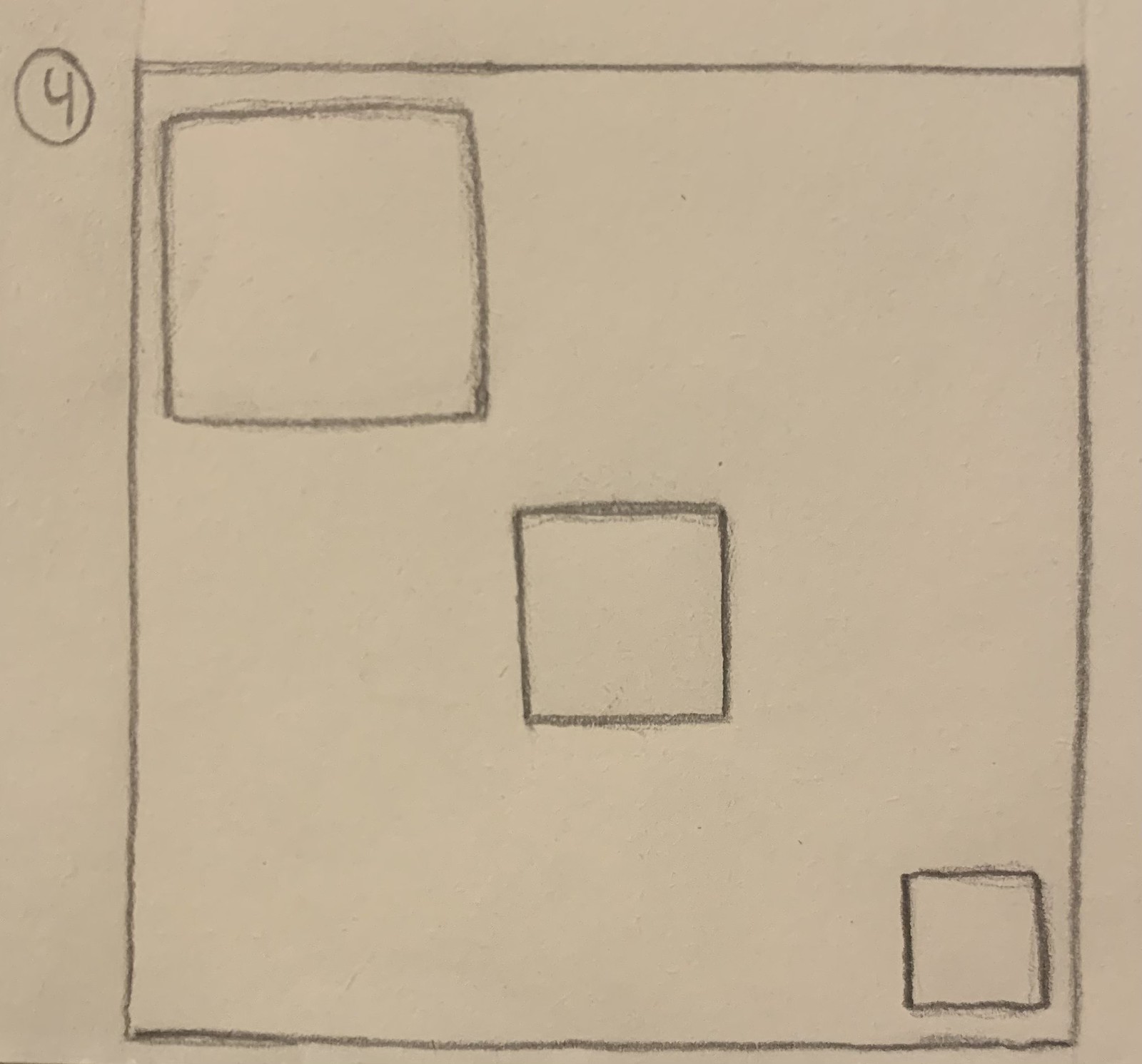This image is a detailed pencil or charcoal drawing rendered on a brown piece of square-shaped paper, measuring approximately 6 to 7 inches on each side. The central focus of the drawing is a large square occupying about 90% of the canvas. In the top left corner of this large square, the artist has inscribed the number '4' within a circle. 

Within the boundaries of the large square, there are three smaller squares aligned diagonally from the top left to the bottom right. The first square, positioned in the top left corner, appears to be around 1.5 inches by 1.5 inches in size. The second square, situated roughly at the center of the large square, measures about 1.5 to 2 inches on each side, making it slightly larger than the first. The third square, located in the bottom right corner, is about half the size of the second square. These nested squares decrease in size progressively as they move from the top left to the bottom right.